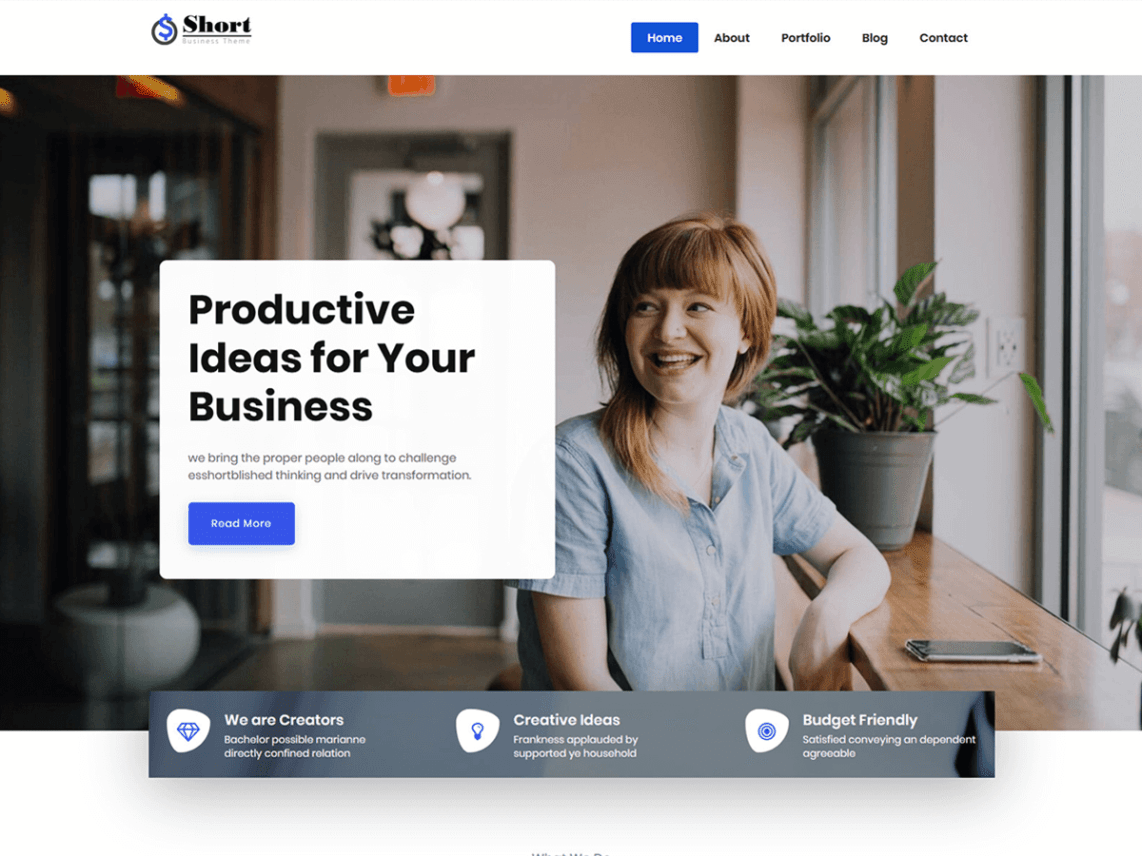The website screenshot features a professional layout. In the top left corner, slightly indented, the business name "Short" accompanied by a logo is visible. Positioned a bit off-center to the right, there are clickable navigation links labeled Home, About, Portfolio, Blog, and Contact.

Dominating the page is a central image of a woman seated at a bar-height table. She has reddish hair and is dressed in a light bluish-gray short-sleeved button-up shirt. Her left elbow is resting on the tabletop, and her phone is positioned in front of her. A plant is also placed on the table behind her. The background wall includes a mirrored section and additional plants.

Overlaying this background, the text reads: "Productive Ideas for Your Business. We bring the proper people along to challenge established thinking and drive innovation." Below this, a clickable button invites users to "Read More."

Towards the bottom of the image, another overlay contains a rectangle with the texts "We Are Creators" and "Creative Ideas and Budget Friendly." Although the print underneath these headings is small and hard to decipher, it consists of several sentences providing additional information.

The foreground reveals large glass windows, suggesting that the setting may be a storefront. This composition creates a professional and inviting atmosphere aimed at engaging website visitors.